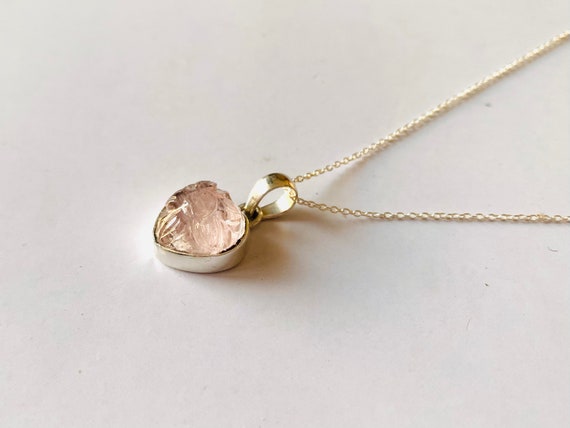This photograph showcases a delicate piece of jewelry displayed on a stark white backdrop. The central focus is a simple pendant with a heart-shaped, clear stone that has a subtle pink hue. The stone, approximately half an inch thick, is encased in a gold outline with a white border. This pendant is elegantly attached to a fine gold necklace, featuring small links and an additional loop adjacent to the pendant. The white background enhances the pendant’s prominence, ensuring that it stands out sharply in the image. The photograph is devoid of any text, people, animals, buildings, or vehicles, maintaining an exclusive focus on the necklace itself.